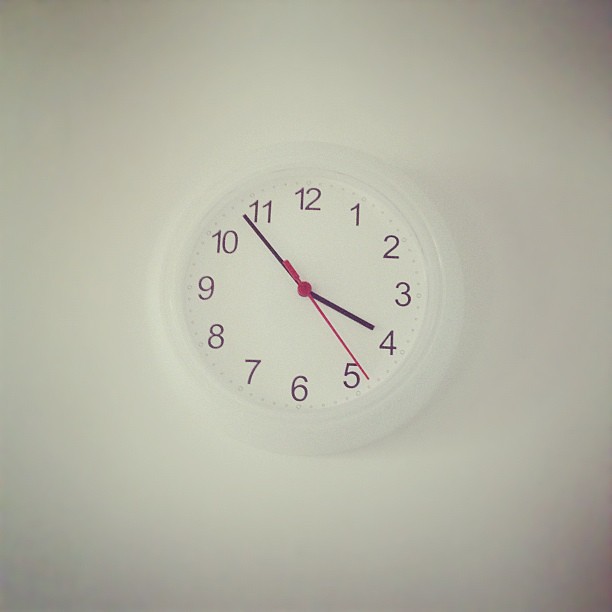The image features a photorealistic depiction of a pristine white wall with subtly shadowed corners that create a gradient effect, drawing the viewer's attention to the center. Mounted on this wall is a minimalist white clock. The clock's face is adorned with sleek black numbers in a standard clockwise arrangement, starting from 12 at the top and proceeding numerically around to 11. In-between each number, small, darker white dots mark each minute interval, adding precision to the design. At the heart of the clock, three hands mark the time: two black and one red, contrasting sharply against the white background, making them easily distinguishable. The overall composition exudes simplicity and clarity, emphasizing the clock's functional elegance.